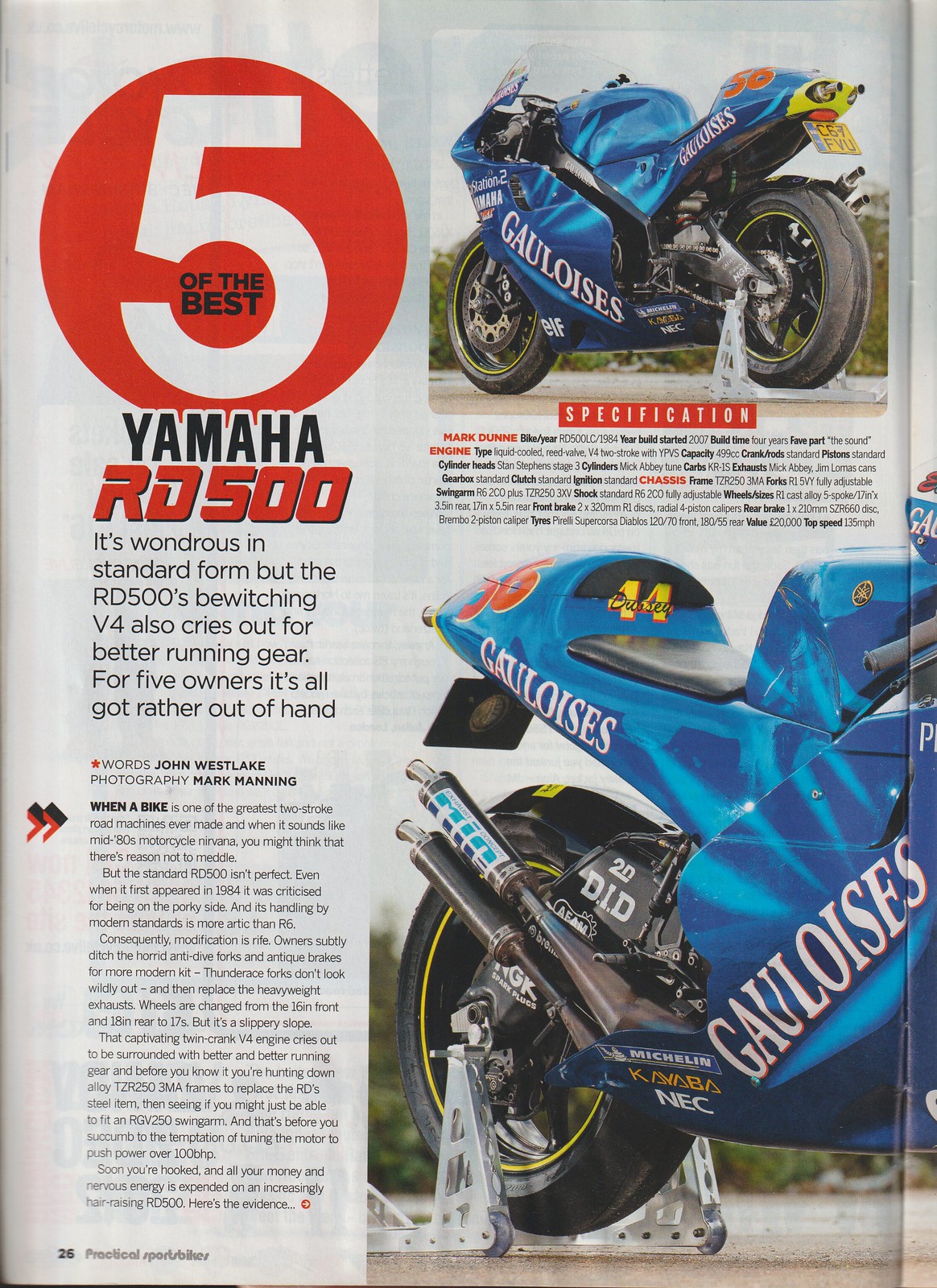This interior page of Practical Sport Bikes magazine, open to page 26, features a detailed article titled "Five of the Best Yamaha RD500." The prominent red circle graphic with a large white "5" and the text "of the best" artfully integrated, introduces the theme of the article. Highlighted is a highly customized blue Yamaha RD500 racing motorcycle, bearing the racing number 56 in red and notable for its shiny finish. Sponsored by Galloises, this bike showcases a custom yellow spot near the exhaust and meticulously detailed modifications. Built and owned by Mark Dunn, who spent four years crafting this machine, his favorite aspect is the distinctive sound it produces. Accompanying the article are two photographs: one showing a three-quarter rear view and another close-up of the side and seat, where features like the custom work on the exhaust and chassis are visible along with the number 44 in yellow near the seat. The article discusses the allure of the Yamaha RD500 in its standard form and the extensive customizations made by enthusiasts like Dunn to enhance its performance.